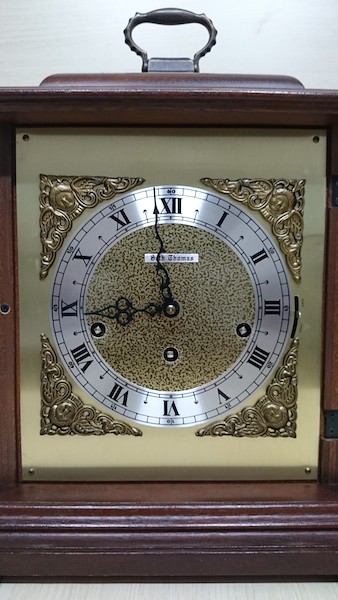This photograph captures an exquisite timepiece housed within a finely crafted wooden box. Atop the box is a small, rounded handle with a silver finish, adding a touch of elegance to the piece. The clock inside features a sophisticated silver and gold color scheme, with its face displaying the time in Roman numerals. The hands of the clock indicate that the time is approximately 8:58 or 8:59. Surrounding the rounded clock face is a square frame adorned with intricate gold metalwork. The background of the clock face presents a unique blend of gold and silver tones, creating a luxurious and timeless aesthetic.